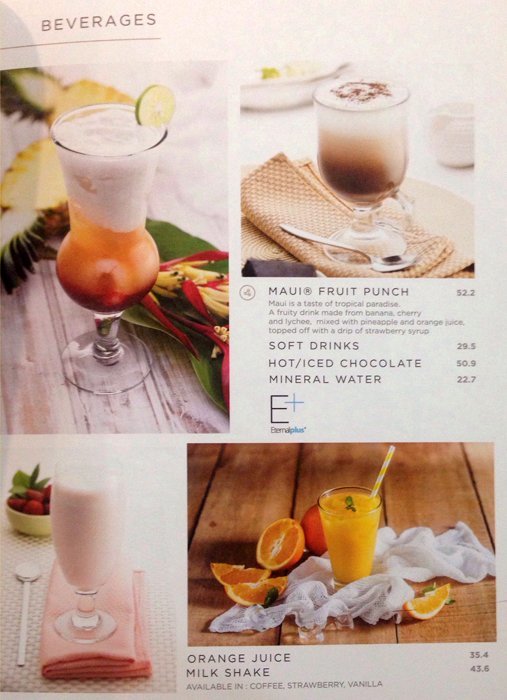This image is a detailed snapshot of a menu showcasing various beverages, set against a white background. At the top left, the heading "BEVERAGES" is bold and underlined. Below this heading is a photo of a tall glass with a frothy white top, an orange layer beneath, and a darker red bottom. This drink is garnished with a slice of lime on the rim, with additional decoration of halved pineapple and flowers in the background. To its right, there is an image of a coffee-based drink in a cylindrical, rounded glass, layered in white, light brown, and dark brown hues, topped with cocoa powder, set on a white napkin with a spoon.

The menu text below the images describes "Maui Fruit Punch" as a "tropical paradise," containing banana, cherry, lychee, pineapple, and orange juices, finished with a drip of strawberry syrup, priced at 52.2. Other beverages listed include soft drinks at 29.5, hot/iced chocolate at 50.9, and mineral water at 22.7. Below these listings, the text "E Eternal Plus" in black letters with a blue plus sign appears.

At the bottom, two more photos are included. On the left, a pink milkshake in a tall glass sits on a long folded napkin with a long spoon beside it, with a background of strawberries in a yellow bowl. The milkshake is offered in flavors like coffee, strawberry, and vanilla, priced at 43.6. On the right, a glass of fresh orange juice is shown, complete with a white and yellow striped straw and surrounded by orange segments, priced at 35.4.